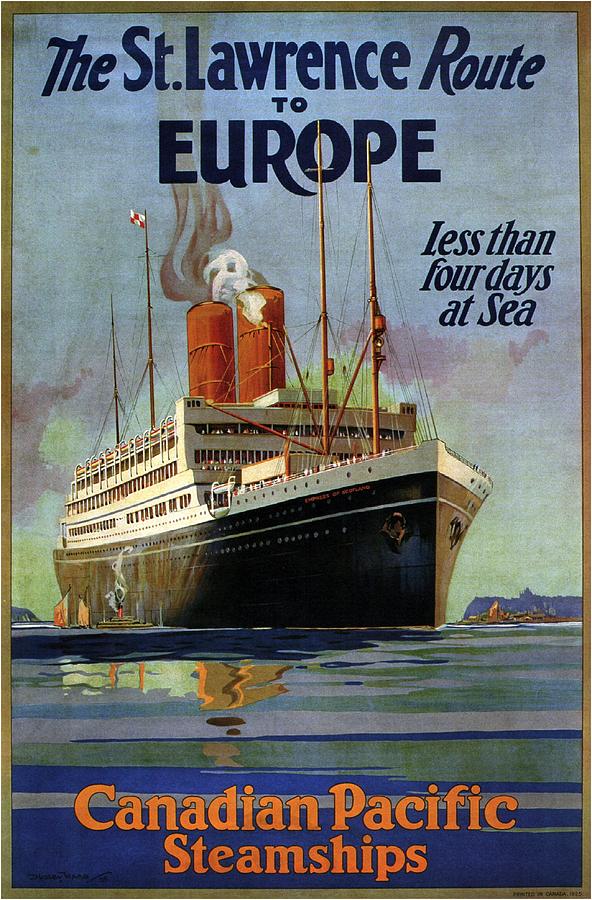The image is a large, vivid poster advertising Canadian Pacific Steamships. Dominating the scene is an artist’s rendition of a colossal steamship, reminiscent of a smaller Titanic, characterized by its black hull and white decks. The ship features striking orange smokestacks emitting smoke, accompanied by various riggings and towering masts, both fore and aft. A red and white checkered flag graces one of the masts. The scene captures the vessel as it seemingly sails into a bay or harbor, with the serene water below reflecting the ship's grandeur.

The backdrop includes a watercolor sky painted in shades of blue and gray with purplish clouds. Tiny figures of people populate the deck and balcony areas, suggesting activities related to either embarking, disembarking, or merely stopping en route. Smaller vessels, including a notable tugboat beside the steamship, highlight the scale of the main ship as they navigate the calm waters, which mirror the surroundings like glass.

The top of the poster proclaims, "The St. Lawrence Route to Europe. Less than four days at sea," in dark blue letters integrated seamlessly into the sky. At the bottom, bold orange letters spell out "Canadian Pacific Steamships," solidifying the historic and promotional nature of the artwork. The poster, imbued with a vibrant color palette and clear illustrative quality, encapsulates the allure and majesty of early 20th-century maritime travel.